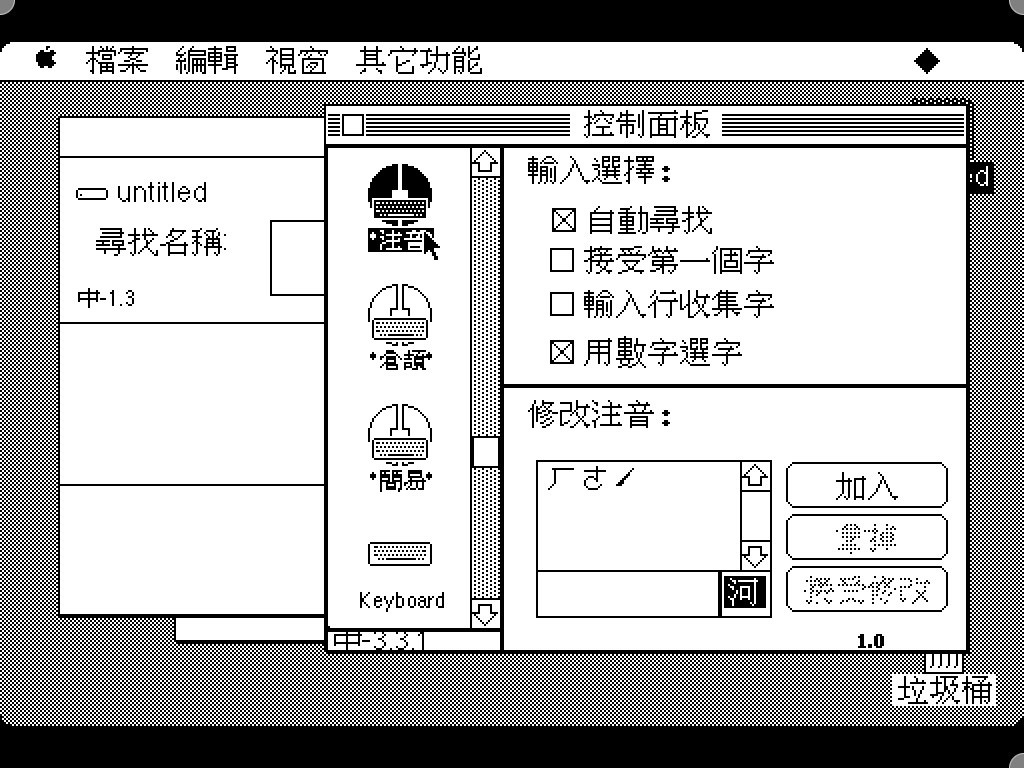The image is a black-and-white screenshot of a computer interface, likely related to a keyboard instructional program or software. The screen features predominantly Chinese or Japanese text, with a layout divided into several sections. At the very top of the interface is a task or menu bar, distinguished by multiple icons, including a logo resembling an apple (though not the Apple Inc. logo), and various symbols written in black font against a white background.

Below the taskbar, the interface is divided into multiple panels. On the left-hand side, there's a tall rectangular menu split into four sections. The top section features the header text "Untitled" followed by script in Chinese or Japanese. Beneath this, there are three evenly divided sections, two of which have no visible text or symbols.

Moving right, there is another menu structured into three sections. The leftmost section within this menu displays four icons, apparently representing keyboards. The middle section contains Chinese or Japanese text within an oblong rectangle. The rightmost section is a larger panel filled with more script in Chinese or Japanese and multiple small rectangular buttons, suggesting various interactive elements or options.

The background of the entire interface features a grayscale dot checkerboard pattern, creating a subtle textured look. In the center panel, clearly labelled "Keyboard," there are illustrations of different keyboards, likely providing visual representations as part of the instructional content. The version of the program, labeled as 3.3.1, is indicated in the middle portion of the interface.